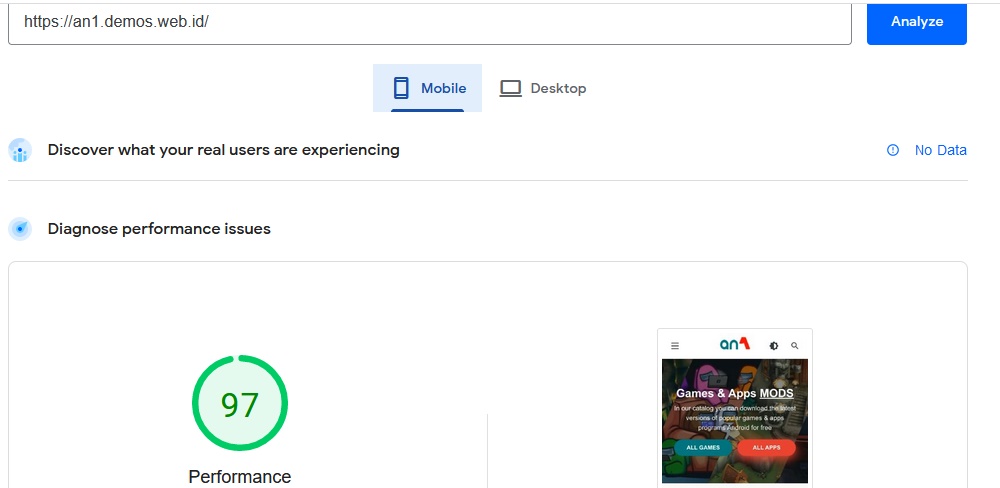The image is a rectangular graphic with a white background, oriented horizontally. At the very top, a black outline box contains the URL "HTTPS://an1.demos.web.id/". To the right of this box, there is a blue button with white text that reads "Analyze".

Moving further down, the image presents two selection options: "Mobile" and "Desktop". The "Mobile" option is currently highlighted with a light blue box around it.

Below these options, a bold statement in black text reads, "Discover what your real users are experiencing." To the far right of this text, there is a blue label that states "No data".

The next line of text says, "Diagnose performance issues," with no additional information to the right.

Enclosed in a gray outline box beneath this section, the left side features a green circle with a dark green highlight along its circumference. Inside the circle is the number "97". The green outline of the circle is nearly complete, indicating high performance. Underneath the circle is the word "Performance."

On the right-hand side within this gray outline box, there is a section labeled "Games and Apps and Mods."